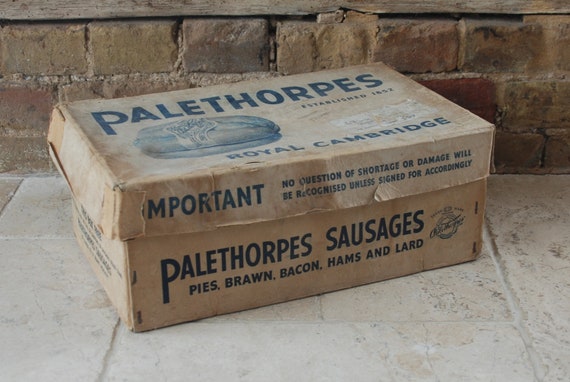The image showcases an old, weathered cardboard box sitting on a tiled sidewalk in front of a brick wall. The rectangular box resembles a large shoebox and appears to have endured the elements. The bricks in the wall behind are varied in color, ranging from lighter brown to reddish hues, with visible grout in between. The ground beneath the box is composed of pale, whitish-gray stone tiles with a matte finish.

The box itself is clearly the focal point of the image and is positioned at an angle, emphasizing its aged condition with worn and faded aspects. It has a detachable lid that is not secured, further indicating its tattered state. The text on the front and top of the box is printed in a dark navy blue font and reads: "Palithorpes sausages, pies, brawn, bacon, hams, and lard." Additionally, the lid bears an image, presumably of bundled sausages, beneath which are the words "Royal Cambridge" and "Established 1852." The photograph appears to be taken outdoors in daylight, providing a clear yet nostalgic glimpse into what seems to be a historic packaging design.